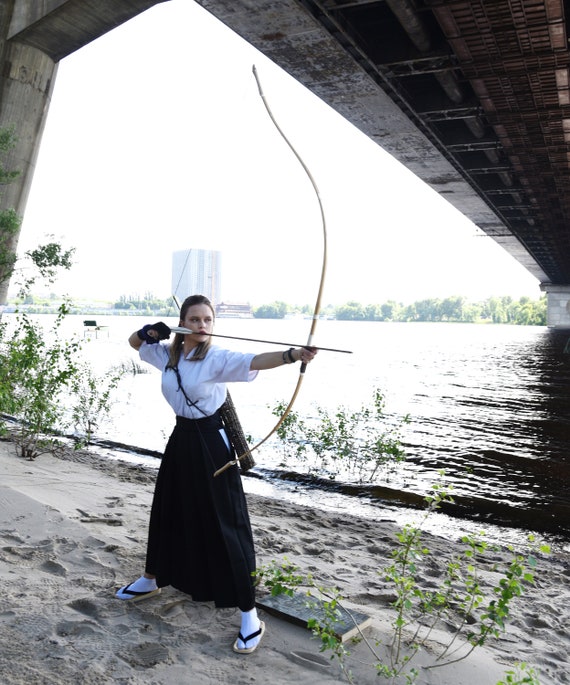In this color photograph, a young Caucasian woman is depicted as an archer. She stands on a sandy riverbank under a concrete bridge, which spans a wide body of water replete with ripples and lined with scrubby plants and trees. The scene is illuminated by daylight, casting a clear sky backdrop. Tucked into her long black skirt, the woman wears a short-sleeved white button-down shirt. She is also noted for her unique footwear—white characteristic socks with sandals.

Her straight, medium-length brown hair complements her serious expression as she draws back an incredibly tall longbow, its tip soaring far above her head. She is captured in a dynamic, slightly twisted stance, facing toward the right of the image, sighting down the arrow which is ready to be released. Accessories include a black glove on her right hand and what appears to be a black bracelet or watch on her left wrist. A quiver is strapped over her shoulder, completing her archer’s attire.

In the background, across the expansive river, stands a building which seems to be a tall skyscraper, possibly sharing the area with other structures. The bridge above her, possibly a railroad trestle bridge, adds an imposing architectural element to the picturesque outdoor scene, merging urban and natural elements harmoniously.